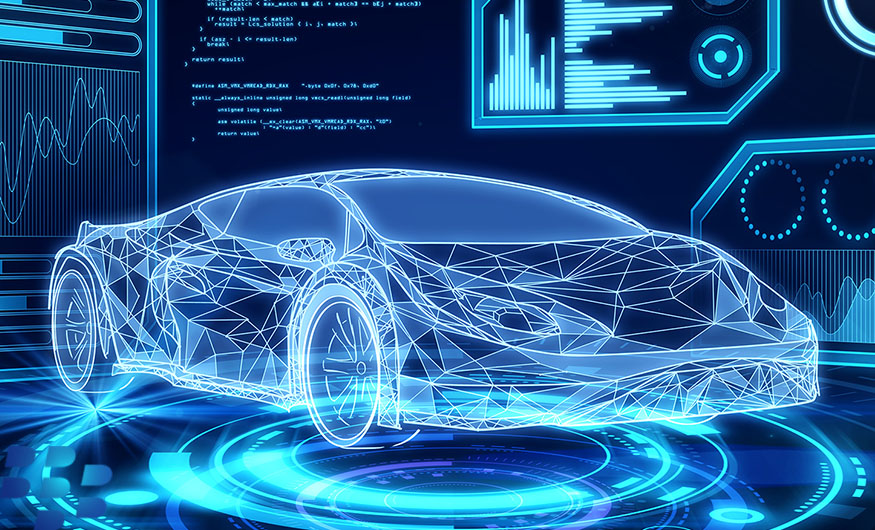The image showcases a digital, computer-generated depiction of a two-door sporty car, intricately designed with irregular triangles giving it a fractal-like appearance. This sleek vehicle is positioned atop what resembles a turntable, suggestive of a dynamic, rotating display. The predominant color scheme features gradients of dark blue transitioning to light neon blue, lending the image a futuristic ambiance.

Dominating the top half of the image is a series of computer-generated visuals. On the far left, wavy lines flow alongside an area of unreadable text, possibly emulating a data stream or analytics display. Adjacent to these elements are several graph-like illustrations: one graph ascends from the bottom to the top, while two others extend horizontally from the left. Central and slightly to the right, a blue and white concentric circle design is nested, featuring a smaller circle within. Below this, an image of two dotted circles—some dots bright blue and others darker blue—further enhances the high-tech feel.

In the lower half, the neon blue rings encircling the base of the car add a final touch to the futuristic, holographic atmosphere, blending seamlessly into the advanced, digital background of the entire image.